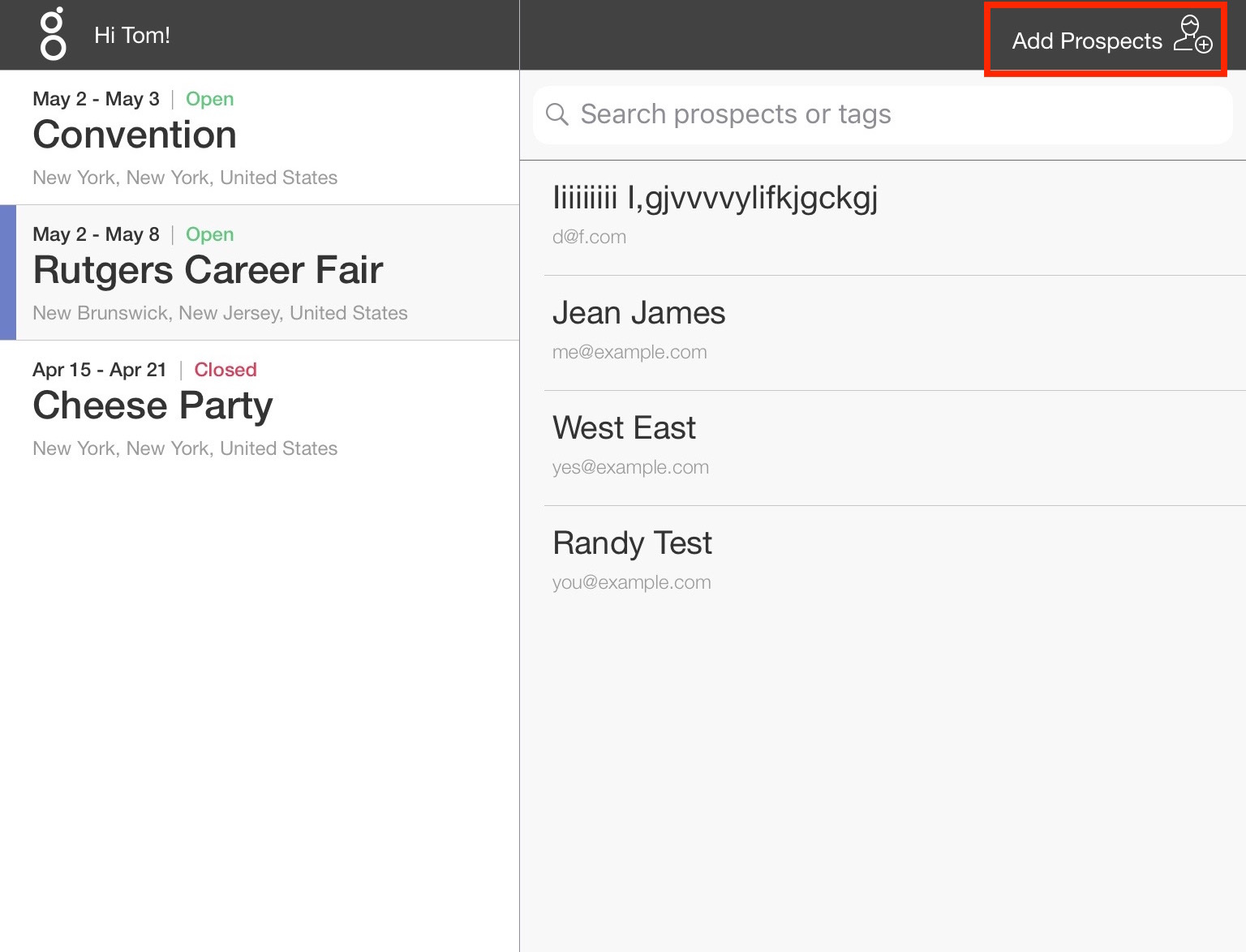The image presents a user interface on a white background adorned with text and various UI elements. At the top, there is a brown header bar featuring the words "High Time" in the upper left corner, accompanied by two circular icons. To the right of this bar, a section contains the text "Add Prospects" alongside an image of a person's upper torso, encased in a red box to highlight it, possibly suggesting an action item.

On the left side of the screen, there is a list of events with the following details:
- "May 2nd to May 3rd, Open" followed by "Convention, New York, New York, United States."
- "May 2nd to May 8th, Open" followed by "Rutgers Career Fair, New Brunswick, New Jersey, United States."
- "April 15th to April 21st, Closed" followed by "Cheese Party, New York, New York, United States."

On the right side, there's a search box labeled "Search Prospects or Tags," which displays search inputs such as "Gene," "James," "West," "East," and "Randy test." Additionally, the top of the screen shows a random assortment of letters and numbers, resembling inadvertent keystrokes.